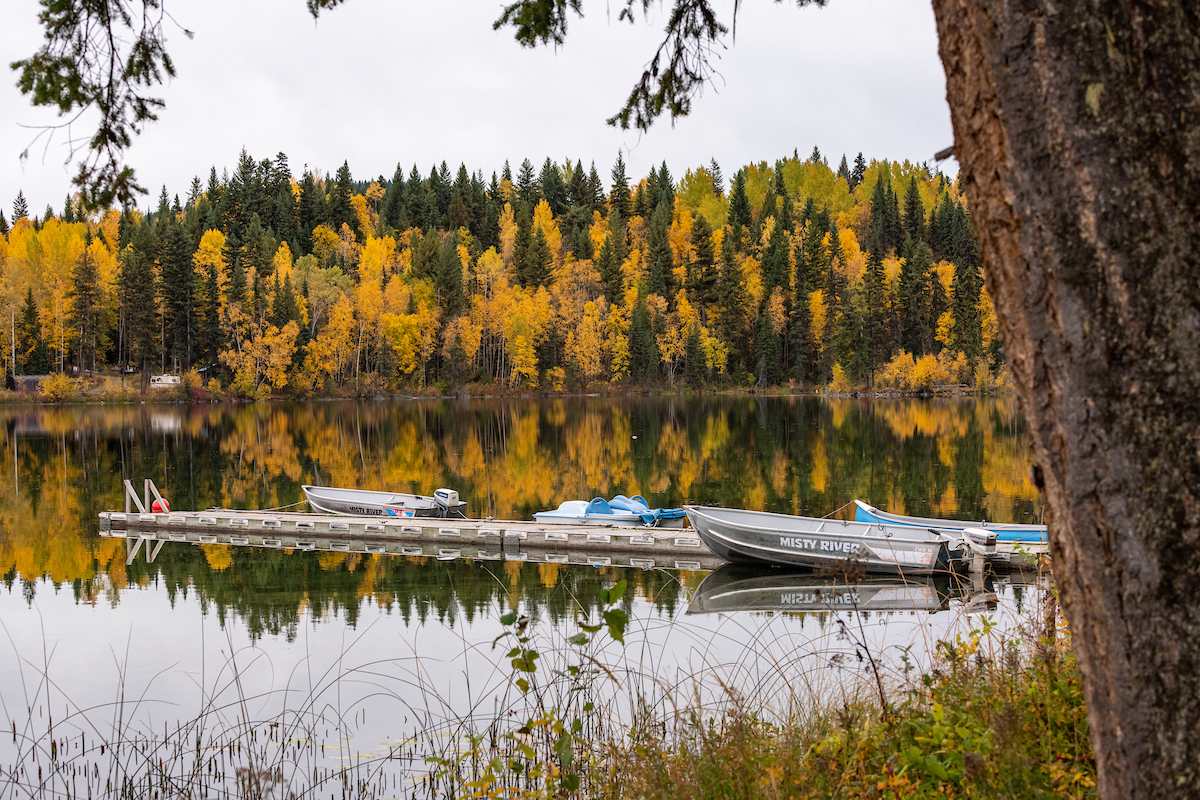The image captures a peaceful lakeside scene in the wilderness, emphasizing the serenity of the natural environment. The lake's calm, brownish waters reflect the surrounding vibrant fall foliage, showcasing an array of green pine trees and yellow-leaved maples. Along the bank, green, yellow, and brown weeds gently rise. Tied to a pier, several boats rest in the water—prominently, a gray motorboat named Misty River. Beside it is a blue canoe and a blue paddle boat. Another motorboat with a gray deck extends out into the lake. To the right of the dock stands a large tree, its trunk brown and leaves partly green, casting reflections in the lake. On the left, beyond the boats, a camper is faintly visible among the dense trees. The top of the image is framed by overhanging leaves, while tall grass adorns the bottom right corner.